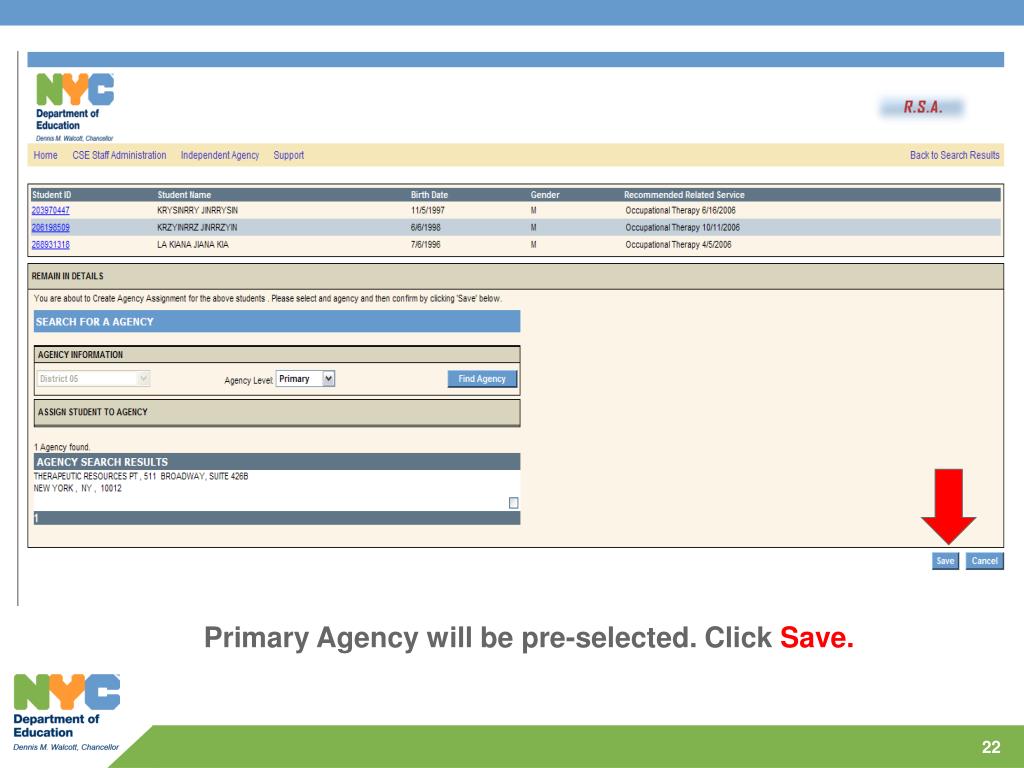This image is a detailed screenshot of a webpage from the NYC Department of Education. At the very top, there's a medium blue horizontal bar that spans the width of the page, followed by a white bar just beneath it, and then another smaller medium blue bar. In the left corner of the uppermost blue bar, the text "NYC Department of Education" is displayed. On the right corner of this same bar, "R.S.A" is written in red font.

Directly below this section, there is a beige-colored bar with blue font housing a navigational menu. The menu items read: Home, CSE, Staff Administration, Independent Agency, Support, and Back to Search Results.

Beneath the navigation menu is a rectangular section featuring a gray bar at the top. The gray bar has white font that labels the table columns: Student ID, Student Name, Birth Date, Gender, and Recommended Related Services. The first row of data in this table displays the following information: 

- Student ID: 203970447
- Student Name: Krysnari Janarsson
- Birth Date: 11-5-1997
- Gender: M
- Recommended Related Services: Occupational Therapy, with a date noted as 6-16-2006.